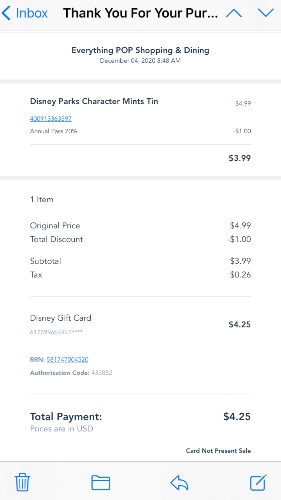Here is a detailed and cleaned-up caption for the described image:

---

The image displays an order confirmation screen from an establishment, viewed on a mobile device. At the top, the screen has a back arrow and the title "Inbox," followed by a "Thank you for your purchase" message. In the top right corner, there are up and down navigation arrows. The background is white, with sections separated by thin gray lines.

The header reads "Everything POP Shopping and Dining," and the transaction took place on December 4th, 2020, at 8:48 a.m. Below this, the purchased item is listed: "Disney Parks Character Mints Tin," originally priced at $4.99. Due to an annual pass discount of 20%, $1.00 was deducted, reducing the price to $3.99.

Further details include:
- Quantity: 1 item
- Original Price: $4.99
- Total Discount: $1.00
- Subtotal: $3.99
- Tax: $0.26

The payment was made using a Disney gift card, amounting to $4.25. An authorization code is included, and the transaction is marked as a "Card Not Present" sale.